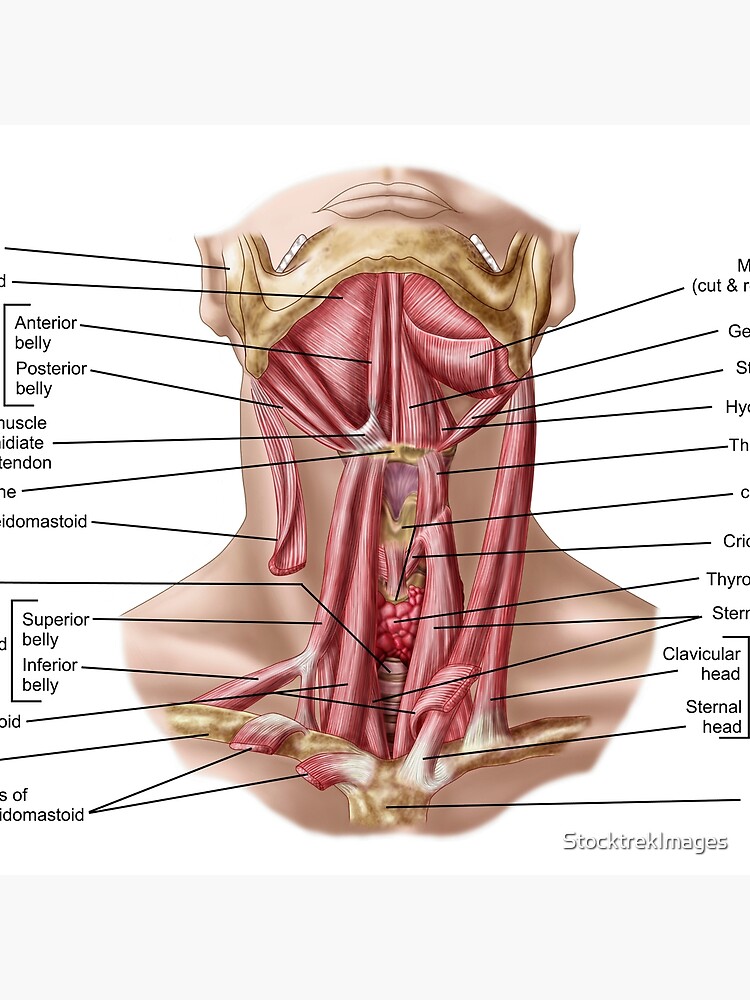The infographic showcases a digitally colored, hand-drawn illustration of human neck anatomy, featuring a detailed view of the throat area, a portion of the chest, and the underside of the chin, all set against a white background. Various muscles, tendons, glands, and other anatomical structures are highlighted, with black lines connecting these parts to corresponding labels, some of which are truncated due to cropping. The legible terms include "anterior belly," "posterior belly," "superior belly," "inferior belly," "clavicular head," and "sternal head." Additionally, the thyroid glands are visibly depicted as bubbly structures within the neck. The bottom right corner contains a watermark from Stock Trek Images. The illustration is complemented by minimalistic red and white shading to indicate the muscles and inner parts of the neck clearly.